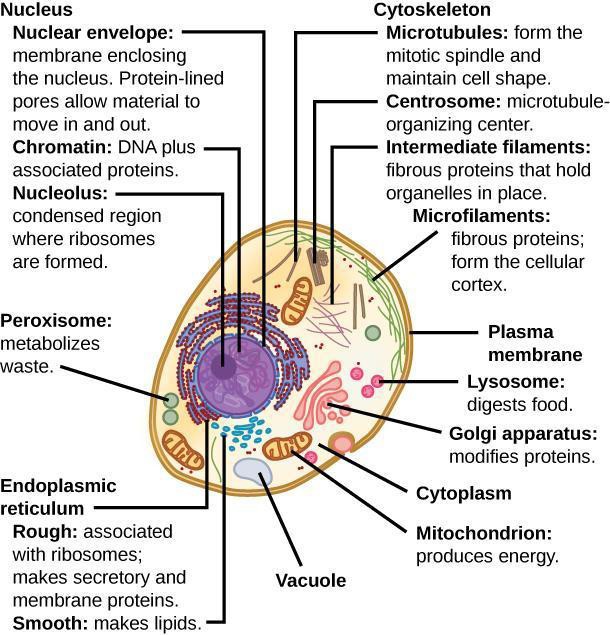In this detailed diagram of a eukaryotic animal cell, the central focus is an oval-shaped structure, outlined in gold and filled with vibrant colors including purple, pink, yellow, brown, and green. At the heart of the cell is the **nucleus**, identified by a blue circle and labeled as having a "nuclear envelope." 

Nearby are two small green circles labeled as **peroxisomes**, described as metabolizing waste. Adjacent to this is the **rough endoplasmic reticulum**, associated with ribosomes and noted for making secretory and membrane proteins, as well as lipids. 

The diagram also includes a gray oval-shaped **vacuole**, essential for storing nutrients and waste. A yellow and gold, peanut-shaped structure represents the **mitochondrion**, the powerhouse of the cell that produces energy.

Surrounding the cell is the **plasma membrane**, which controls the movement of substances in and out of the cell. On the right side inside the cell, there is a small pink, round **lysosome** responsible for digesting food particles.

The upper right section depicts the **cytoskeleton**, including **microtubules** that form the mitotic spindle and maintain cell shape. The cell's structural framework is further supported by an area marked as the **centrosome**, **intermediate filaments**, and **microfilaments**, the latter resembling long strands of grass, identified as fibrous proteins.

This comprehensive illustration captures the intricate components of an animal cell, each meticulously labeled to highlight its function in maintaining cellular activities.